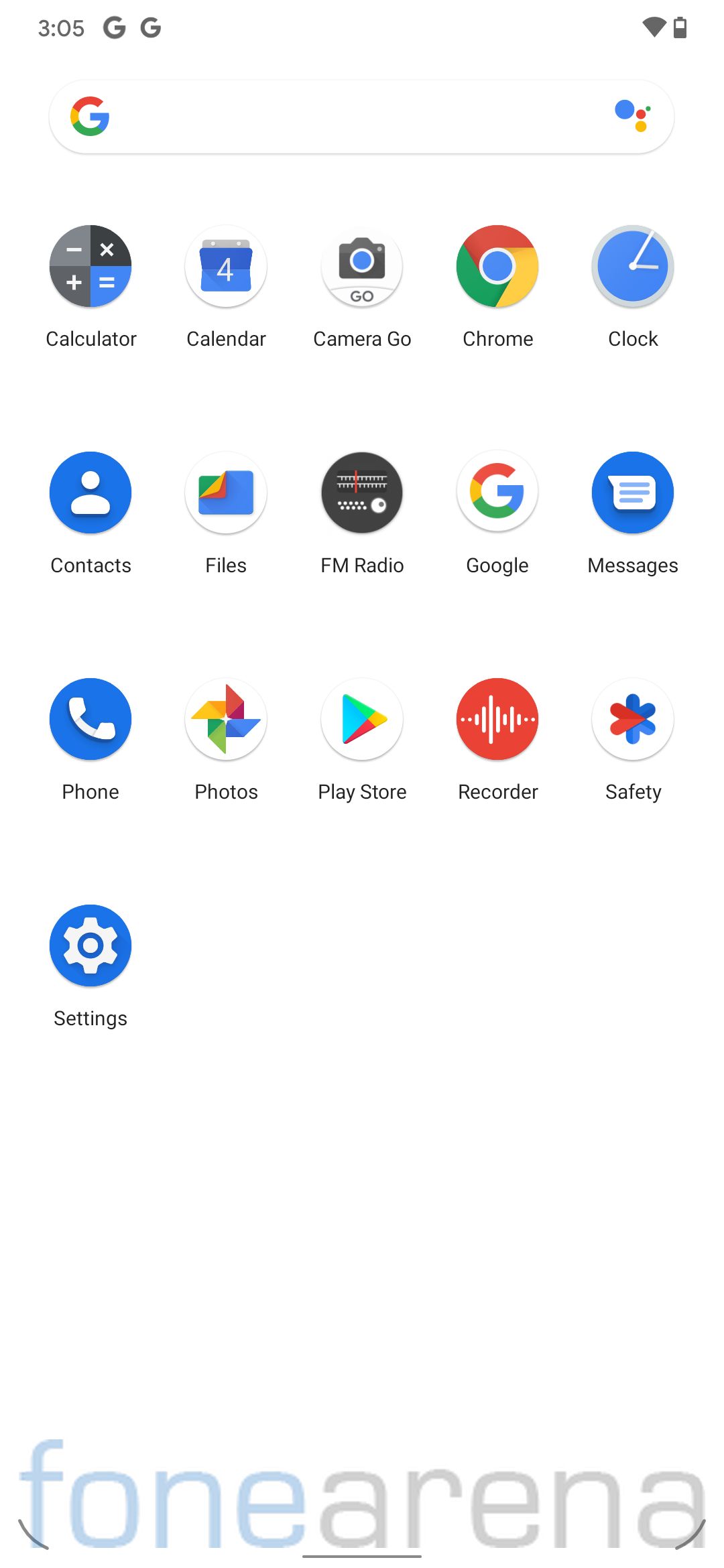A screenshot from a mobile device is showcased with a predominantly white background. At the very top left corner, the time is displayed as 3:05. Directly beneath the time, a Google search bar is prominently featured, adorned with the iconic multicolored 'G' logo in red, yellow, green, and blue. Below the search bar, there are three rows of various application icons arranged neatly. The first row includes the Calculator, Calendar, and Camera Go icons. The second row features icons for Chrome, Clock, and Contacts. The third row displays Files, FM Radio, and Google Messaging. The screen also includes a fourth row consisting of a single icon, which is for 'Settings.'